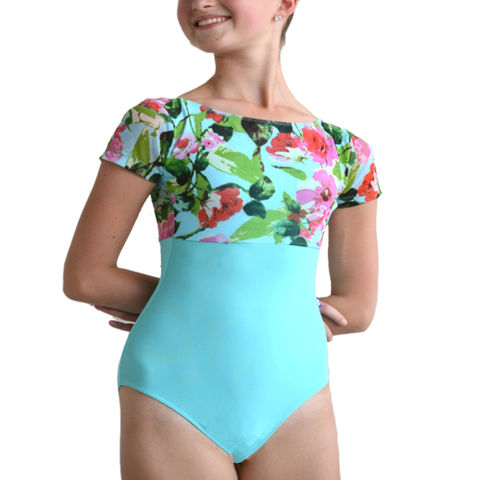The image features a young girl, possibly a preteen, posing against a white background. She is wearing a form-fitting leotard or one-piece swimsuit. The bodysuit has a distinctive design: the bottom portion, spanning from the top of her thighs to her midsection, is a light baby blue or periwinkle color. The top part of the leotard, which includes cap sleeves, is adorned with a bold, vibrant floral print featuring red and pink hibiscus flowers and green leaves set against the same blue background. The girl is facing slightly towards the left, with her hands positioned behind her back, and her face is partially visible, showing up to her nose. She has a smile on her face, adding a cheerful touch to the image. The photo seems to be taken for a clothing website or retailer, highlighting the detailed design of the leotard.